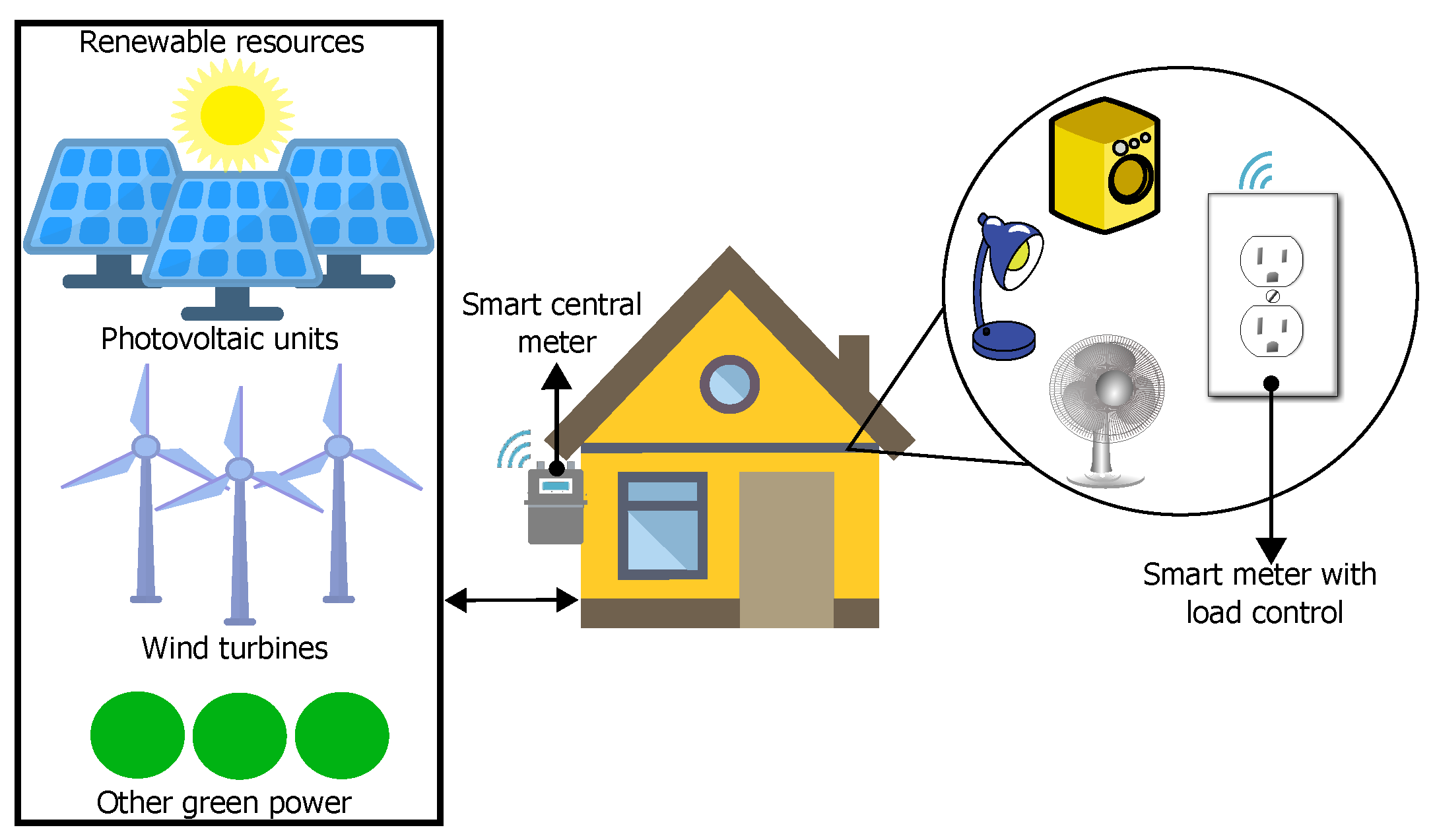This detailed diagram illustrates the process of how renewable energy sources power a home through a smart meter system. On the left side of the diagram, a black rectangular box titled "Renewable Resources" contains images of three solar panels under the sun, labeled "Photo of Photovoltaic Units," three white wind turbines, and three green circles labeled "Other Green Power." An arrow points from these renewable sources to a yellow house, which has a brown roof, brown trim, two windows (a circular one at the top and a square one at the bottom), a rectangular door, and a brown chimney. This house is equipped with a "Smart Central Meter" that connects to an exploded view showing various appliances, such as a lamp, a yellow box with a button, outlets, and a fan. This view, labeled "Smart Meter with Load Control," demonstrates how energy from the renewable sources is managed within the home to power these devices. The smart meter also has a radio signal indicator, suggesting it can communicate or be monitored remotely. The arrows and connections illustrate the flow of energy from the renewable sources to the home's central meter and then to individual devices, emphasizing the efficient and controlled distribution of green power within the home.